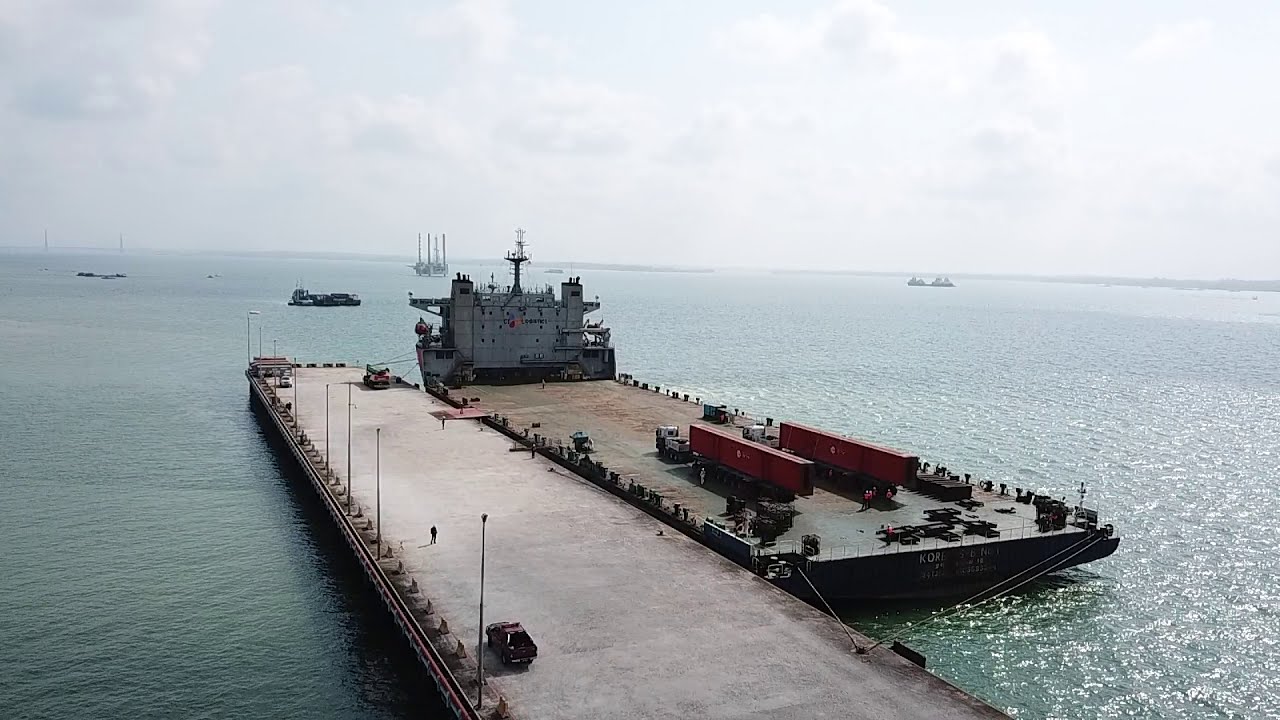This photograph captures a sprawling cement dock extending into a calm, light blue body of water, likely a bay. Centered on this dock is a massive, almost completely flat transportation ship, devoid of most of its typical cargo. The ship has an expansive, wide and long structure with a rusty brown exterior and sports a few orange and red sea crates scattered sparsely on its deck, indicating its capacity to carry hundreds more. The vessel is connected to the dock via a ramp and features a multi-story command center at the front, serving as the navigation and living quarters for the crew. The pier, only hosting this single enormous ship, stretches off the right side of the frame, lined intermittently with light poles and including areas where vehicles and a truck are parked. People can be seen walking along the cement path, adding a sense of scale to the scene. Surrounding the dock, the water remains calm with the horizon revealing several smaller boats and ships floating in the distance under a sky dotted with a few clouds, emphasizing the serene ambiance of the bay.